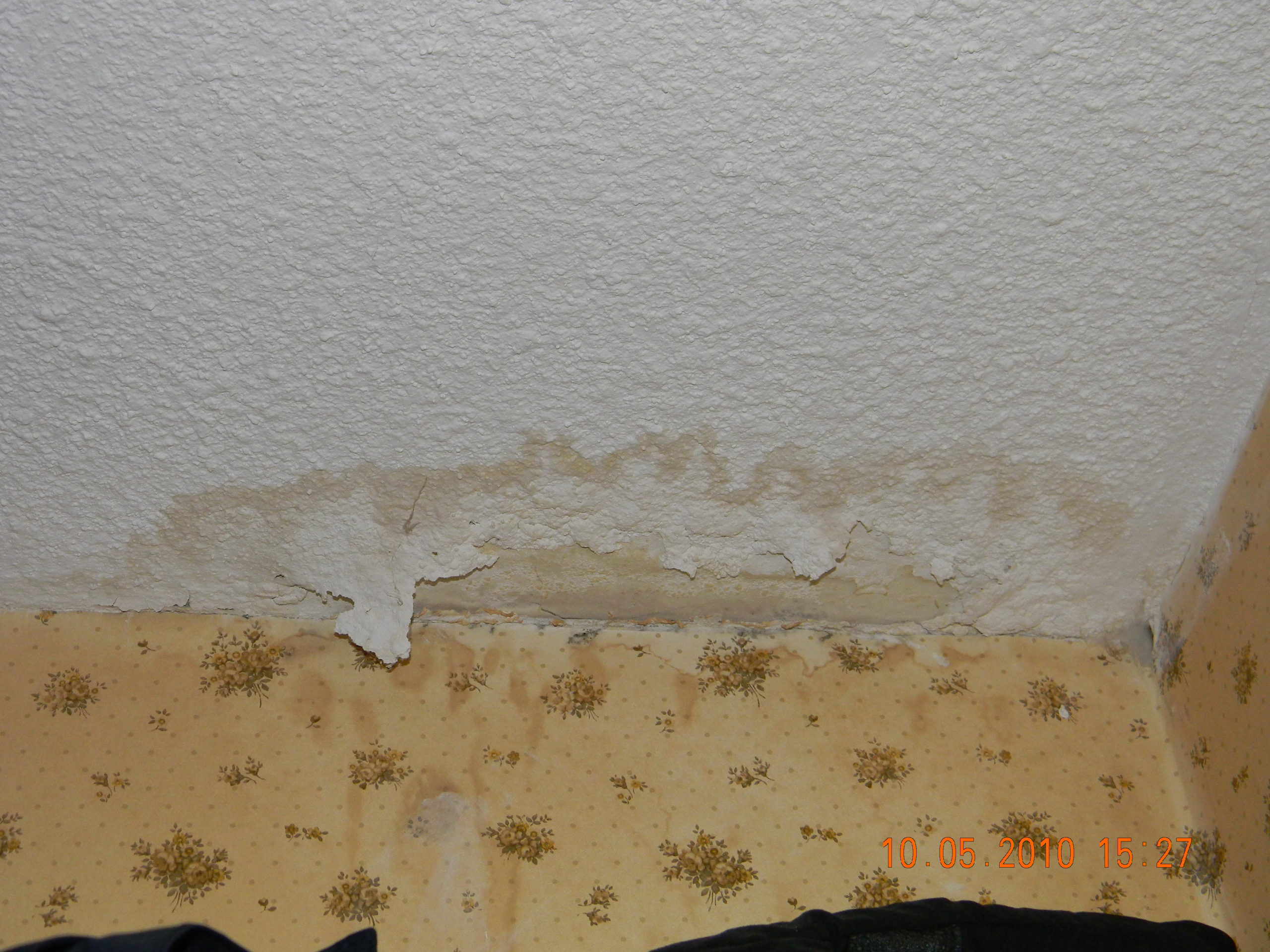This detailed rectangular photo captures a white popcorn-textured ceiling exhibiting significant water damage. The intersection where the ceiling meets the corner of the walls is prominently positioned just below the middle right edge of the image. A considerable portion of the bottom of the image is dominated by a wall, which curves up diagonally toward the bottom right corner. The wallpaper adorning this wall, originally white with patterns of tiny flowers, now exhibits a light brown hue, marred with dark brown and green stains due to the water leak. Noticeable are darker brown streaks descending the wall from the ceiling. The damaged section of the ceiling displays tan watermarks and peeling white paint chips. A timestamp at the bottom right corner reads "10-05-2010-1527," indicating when the picture was taken.